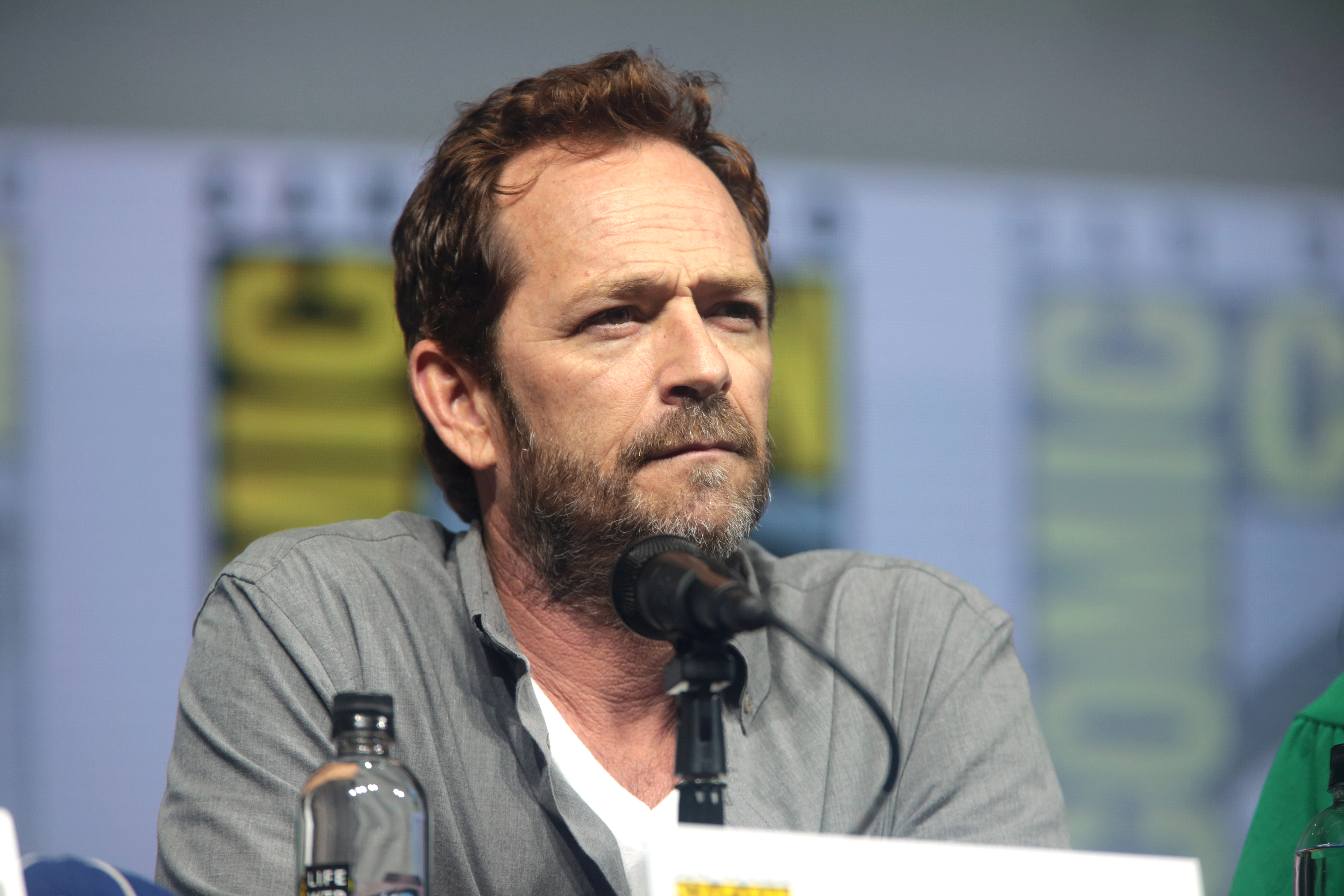An older white man, possibly in his 50s with brown hair and a graying beard, is seated at a Comic-Con event. He is dressed in a gray jacket over a white shirt. In front of him is a microphone, indicating he is part of a discussion or panel. A bottle of water sits on the table to his left. Behind him, the iconic Comic-Con logo is prominently displayed, confirming the event's location. His name placard is visible but partially cut off on the bottom right of the image, making it difficult to identify him. The man appears to be attentively listening, perhaps to a question from the audience.